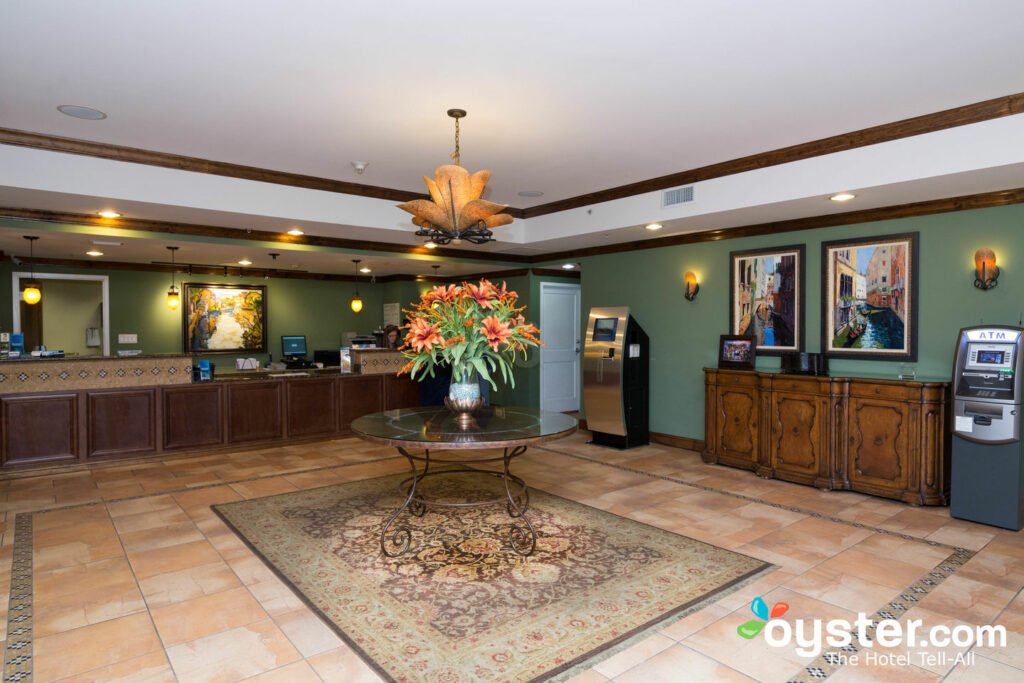This image depicts the lobby of a business establishment, likely a bank or hotel. The floor features brown tile squares with a central rug that boasts a Moroccan-inspired design in brown and tan tones. The walls are painted in an olive green color, adorned with framed artwork. Dominating the center of the room is a round glass-top table with a brown frame and rim, topped with a striking flower arrangement of orange hibiscus-like flowers with long green leaves. Suspended above this table is a chandelier resembling a large orange flower. On the right side of the image, there is an ATM machine, glowing with white light and showcasing a blue interface with a digital screen. Adjacent to it, a long brown counter stretches across the wall, equipped with additional artwork. To the left of the counter stands a silver-fronted machine obstructing a white door. On the left-hand side of the room, the main counter or front desk is positioned, with a lady visible behind it. The expansive room is marked by its open floor plan and meticulous decor, reflected in both the furnishings and architectural elements.